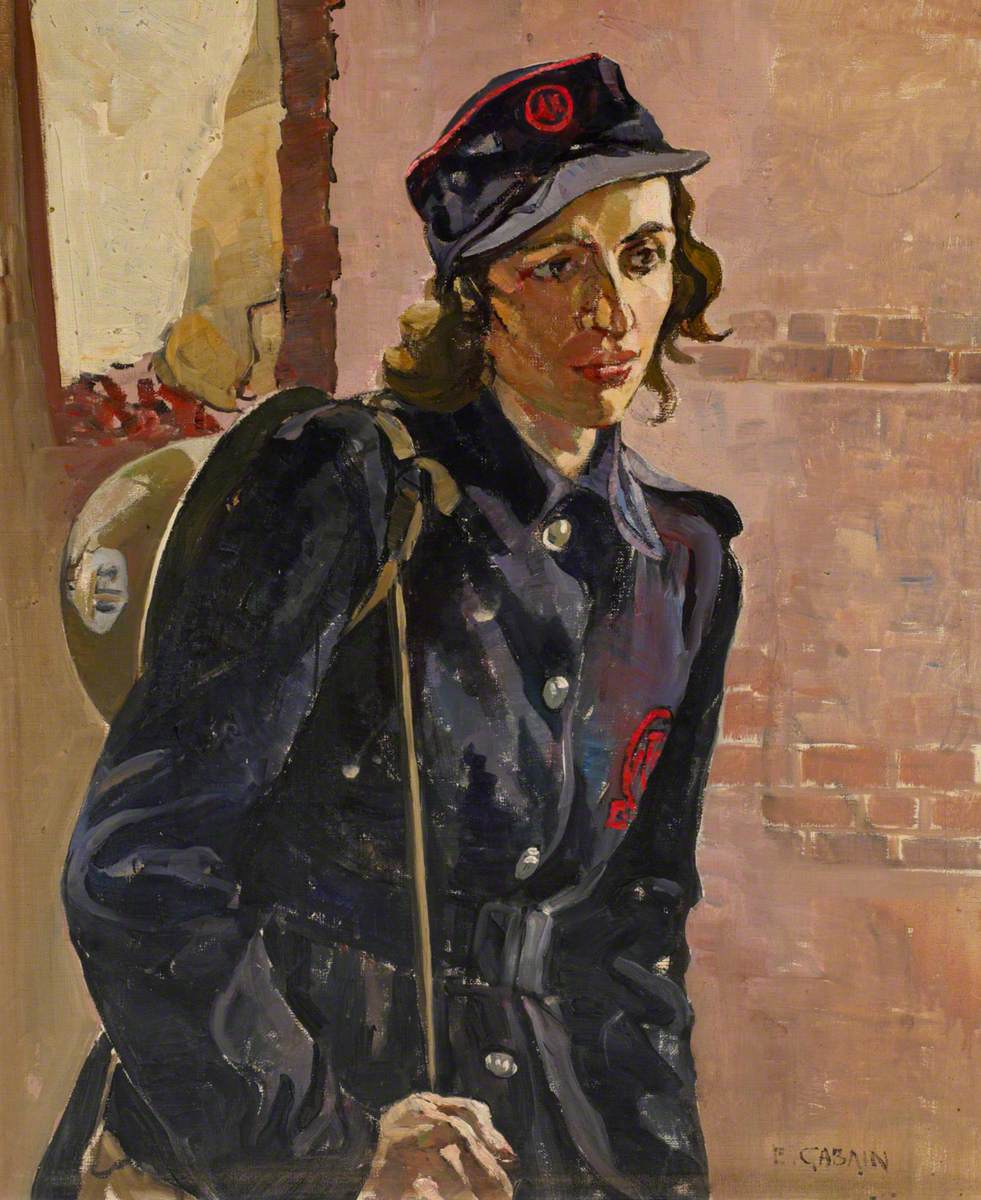This image is a detailed painting featuring a female soldier in a blue uniform adorned with a red patch on the left side of her chest and silver buttons down the front. She is wearing a matching blue cap, also marked with a red emblem. The soldier, with long, curly brown hair, stands in front of a weathered, pinkish-brick wall, which contrasts vividly with the deep blue of her attire. Behind her, the wall has an open window that is devoid of glass. Over her right shoulder, she carries a sandy brown helmet attached to a strap, with a matching colored bag. The scene has bold, yet slightly faded, colors which are distinctly solid and not heavily blended. The painting has an overall lavender and terracotta salmon hue, further enhancing the vividness of the brick and uniform. The piece is almost square-shaped, being slightly taller than it is wide, and features the artist's signature in the lower right corner.